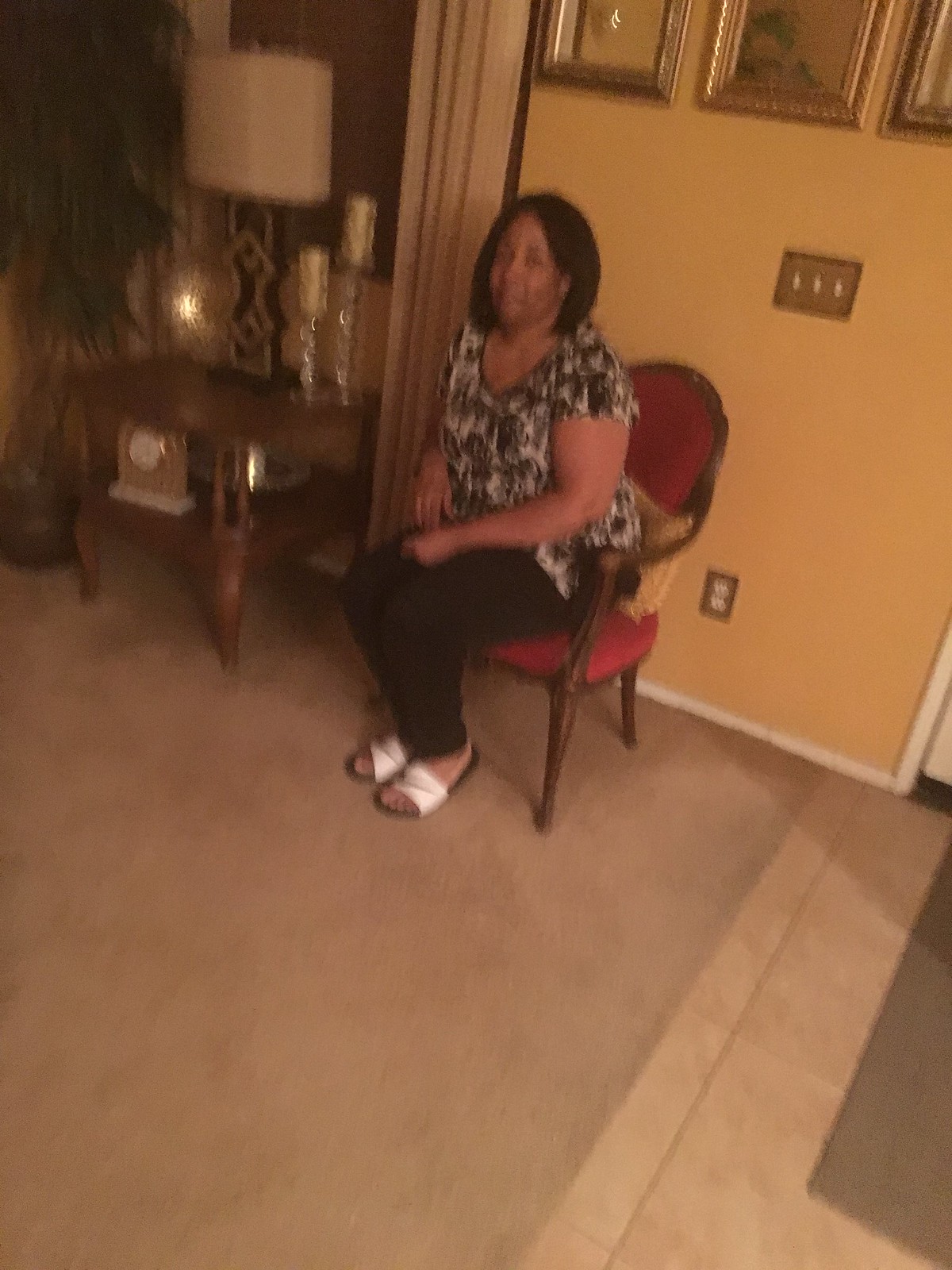In a cozy living room, a woman is seated on a red upholstered wooden chair positioned against a mustard yellow wall. The wall is adorned with three gold-framed pictures and features a three-switch light switch, as well as an outlet near the bottom. The woman, who has chin-length black hair and a darker tan complexion, is dressed in a short-sleeved black and white blouse, black pants, and white slide sandals with a black mark. To her left sits a table holding a lamp with a shade, a small clock, and two candles in candle holders. The room’s floor transitions from a cream-colored rug to a light tan tile, with a dark gray mat also visible. The photograph, taken in portrait mode, captures the serene atmosphere of the space despite some blurriness.